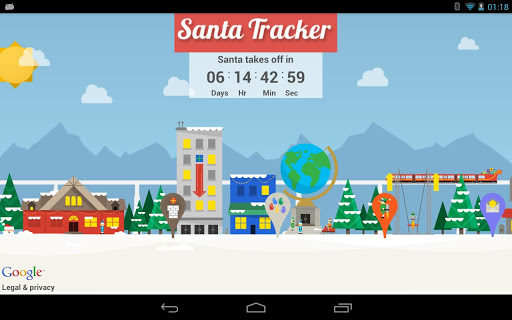Screenshot of the Santa Tracker website interface. The screenshot features a modern, festive design with a black background on the top and bottom sections, adorned with gray buttons. Important information such as the time, battery percentage, and Wi-Fi status are displayed in a light blue font.

At the top center of the image is a prominently displayed red box with the title "Santa Tracker" in white font. In the bottom left corner of the screenshot, the word "Google" is shown in its characteristic multicolored logo. Beneath it, in black font, are the words "Legal" and "Privacy."

Below the "Santa Tracker" title, a countdown timer is presented in a light bluish-white box with black text. The timer indicates the time left until Santa's takeoff, showing "6 days, 14 hours, 42 minutes, and 59 seconds" at the moment the screenshot was captured.

The background features an animated winter town scene. Snow-covered ground and triangular snow-topped trees dominate the foreground, creating a festive landscape. The backdrop includes mountains in darker bluish-gray hues, under a dusty blue sky with drifting clouds. The sun is partially visible on the left side of the sky, slightly obscured by a cloud.

Various buildings of different sizes and shapes, including one capped with a globe, populate the town. Pins are scattered around, suggesting an interactive map element. There are small figures dressed like elves scattered across the scene, bringing the setting to life. Notably, Santa Claus himself is visible in the snow, with his head poking out near the left side in front of a green tree.